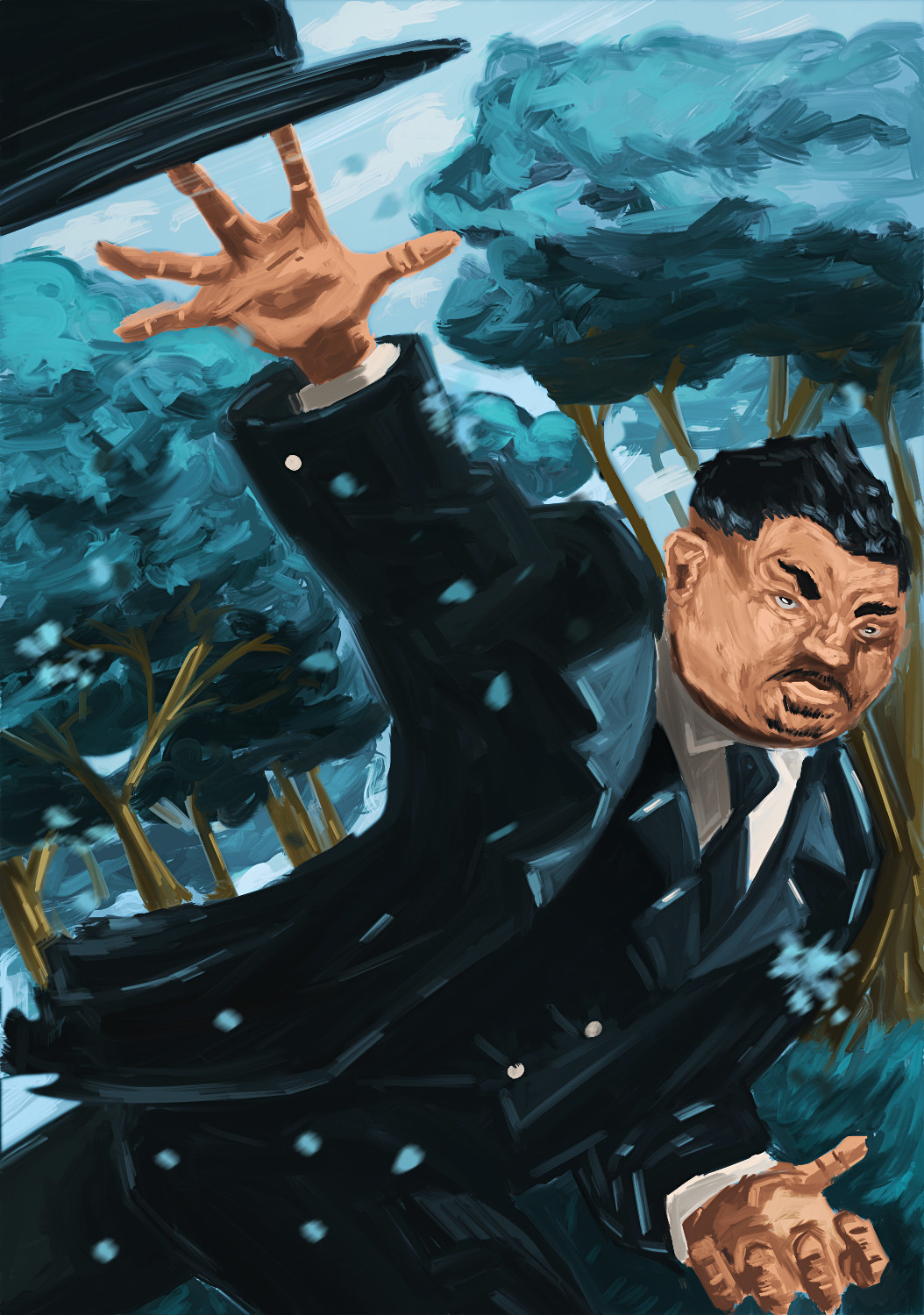This painting features Oddjob, the iconic Bond villain, rendered in a dramatic action-packed style reminiscent of an animated comic book. Oddjob, who appears to be in his 40s or 50s with distinctive black hair, pronounced eyebrows, a small black mustache, and a tiny goatee, is pictured in a tense and dynamic moment. He has tanned, darker skin and piercing blue eyes, adding to his menacing appearance. Dressed in his signature outfit, he wears a black suit complete with a white button-up shirt, a black tie, and a black vest.

Oddjob is captured mid-action, winding up to throw his infamous black, wide-brimmed top hat as a weapon. His right arm is outstretched above him, fingers spread wide, while his left arm is bent, with his hand clenched into a fist closer to his body. The tilt of the painting adds to the sense of movement, making it appear as if he is either running or bracing himself against a strong wind, suggested by the subtle tilt of the image.

In the background, there are tall, green trees with branches swaying, further emphasizing the windy environment; you can even see small dots of debris being blown around. The trees are painted in rich, deep greens and browns, which contrast sharply with Oddjob's dark attire, creating a vivid and intense scene. His top hat is seen in the left corner of the painting, suggesting that he has just released it towards an unseen target. The overall color palette of the image is dark and moody, with deep blues and blacks, enhancing the sense of urgency and action.